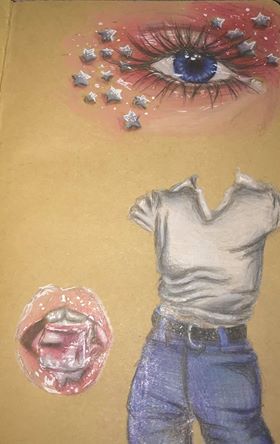This intricate drawing features a captivating, almond-shaped eye at the top, serving as the background. The eye is a mesmerizing shade of blue, framed by long, lush lashes and embellished with star appliques that add a whimsical touch. The surrounding eye makeup is a soft, pink hue, enhancing the eye's natural beauty.

Below this enchanting eye, the drawing displays disembodied clothing, specifically a white t-shirt paired with blue jeans and a black belt, suggesting a feminine figure without depicting an actual person. To the left of this attire, there's an open mouth, possibly containing a vague object that is difficult to discern. The entire composition is rendered in soft pastels, creating a visually appealing and dreamlike portrayal of a female form.